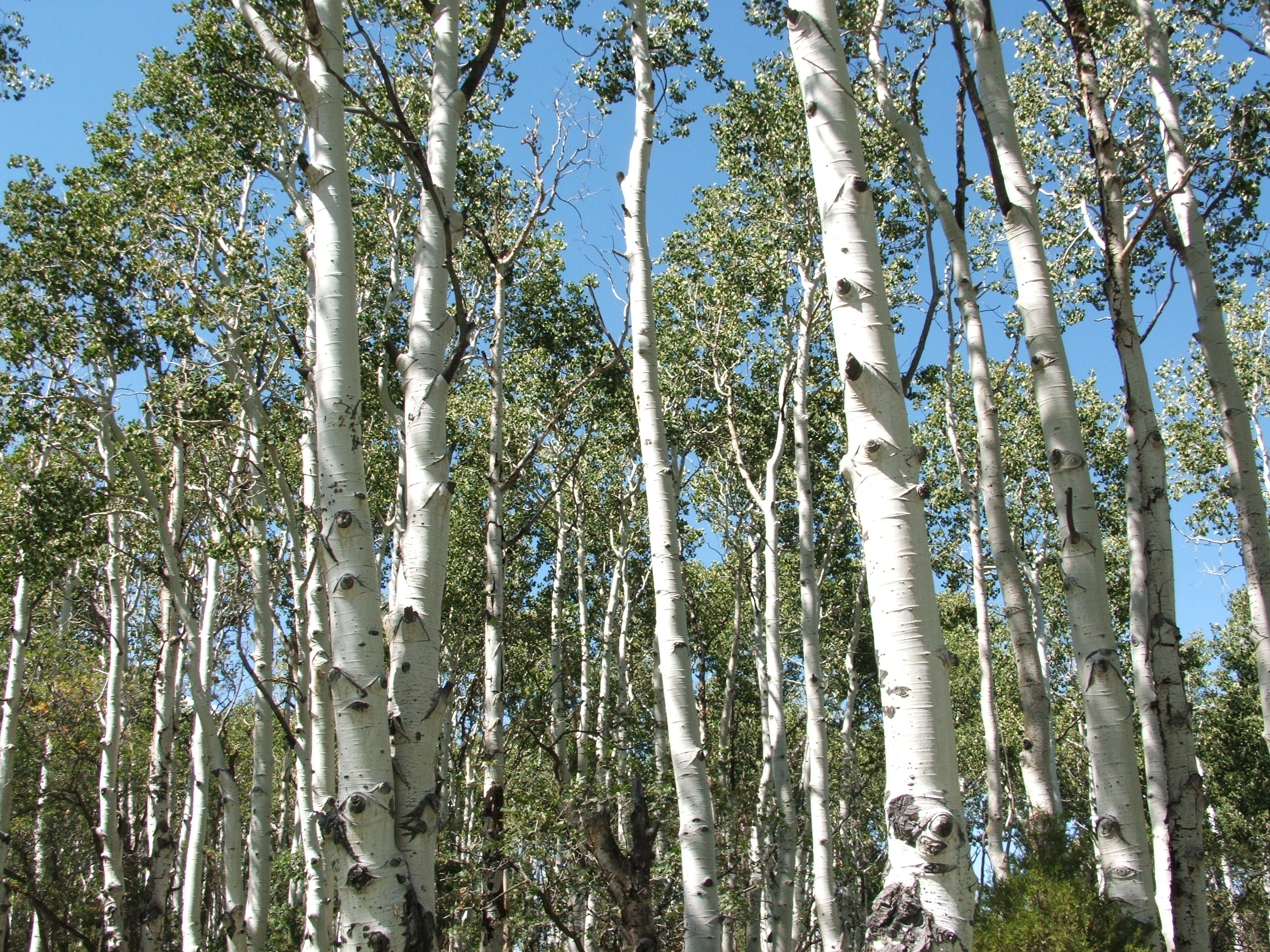The image depicts a bright, daytime scene of a serene birch forest characterized by tall, slender trees with distinctive white bark. Many tree trunks exhibit marks where branches once were, although some green-leaved branches still remain. These leafy branches are primarily concentrated at the tops of the trees, while their slender trunks extend straight from the forest floor to the sky. The vibrant blue sky in the background is clear and cloudless, adding to the tranquil atmosphere. The forest floor features a mix of smaller trees and shrubs, contributing layers of green hues to the overall palette. The colors in the image range from the various shades of green and the white and off-white bark to the grays and browns of the tree trunks. The trees are not densely packed, allowing for glimpses of the clear sky above and creating a sense of depth and openness within this natural setting.